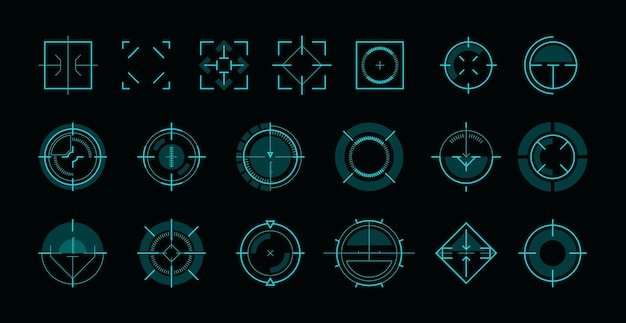On a stark black background, a grid of 18 intricate reticle designs is displayed in three rows and seven columns. These vivid, teal-colored reticles resemble targeting scopes often seen in first-person shooter games. While most are circular with complex line patterns, some are square, particularly in the top row. Notably, the last two designs in the top row are round. The middle row exclusively features circular reticles, and the bottom row includes predominantly circular shapes with one unique diamond-shaped design. All these reticles are distinct yet cohesive in their purpose of aiding target acquisition, showcasing elaborate and varied configurations.